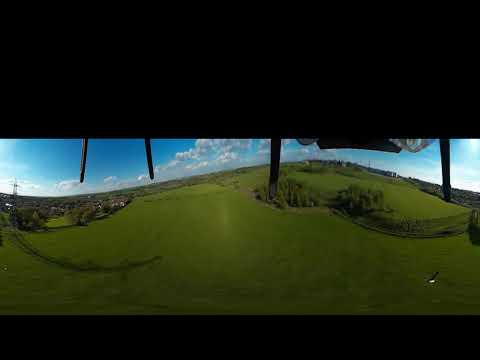The image is an aerial shot taken from an unknown aircraft, possibly a helicopter, capturing a hilly, green landscape. The foreground features a prominent grassy hill, surrounded by scattered bushes and trees. The landscape stretches into the distance where a small town is visible. The photo, taken on a sunny day with some clouds in the sky, includes a wide variety of colors such as green, blue, white, gray, black, and brown. The sky occupies the upper part of the frame, which is partially obscured by a large black overhang or border, suggesting the photo was taken from within a vehicle or building. The frame also includes borders at the top and bottom, with the top border being notably larger.  Additionally, there is a pole visible on the far left side, enhancing the contextual setting of a serene, somewhat rural, outdoor location, possibly observed from a few thousand feet above ground level.